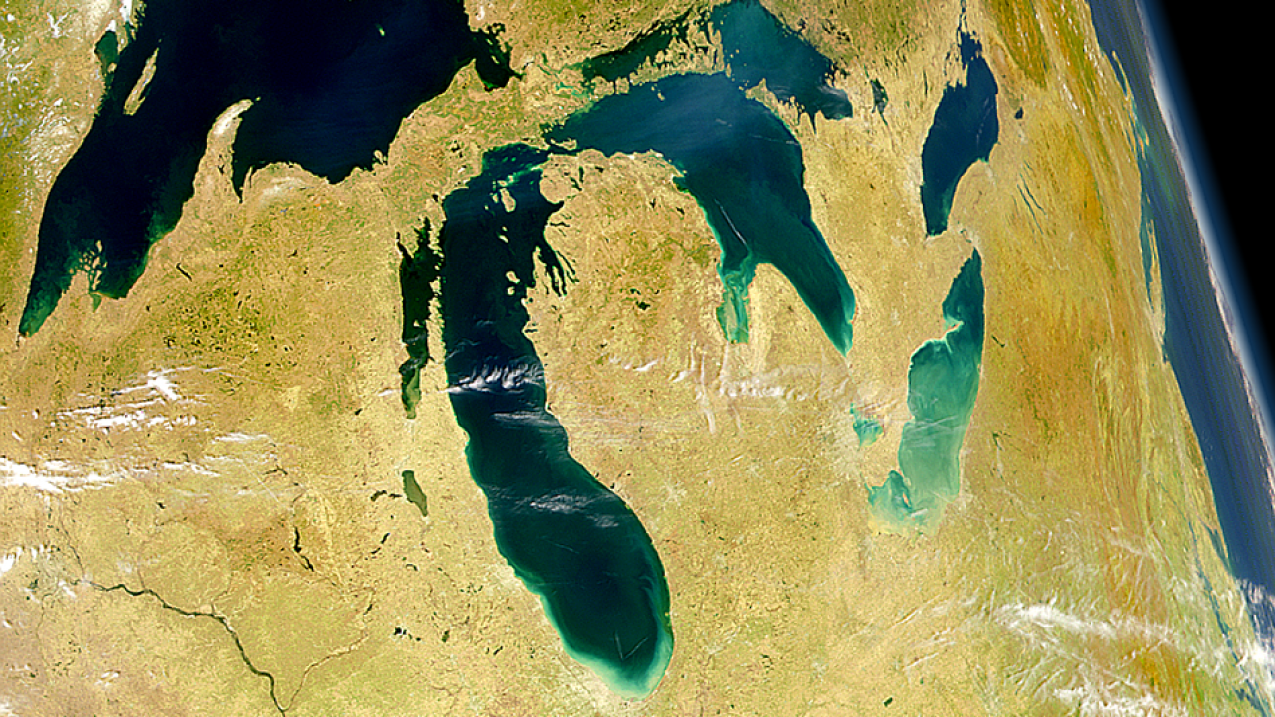The image depicts a stunning view of Earth from space, focusing on a section that prominently features the upper Midwest region of the United States. On the right-hand side of the image, the curvature of the Earth is visible, highlighted by a hazy white glow that contrasts against the expansive blackness of space. The left portion of the image showcases the land mass of the Midwest, with notable emphasis on the state of Michigan, surrounded by the other states like Illinois, Wisconsin, Indiana, Ohio, and New York.

The terrestrial area features a diverse palette of colors, with the land presenting goldish, rocky, and sand-like textures that suggest a desert-like environment. Interspersed among the land are bodies of water, including the Great Lakes, which display a gradient of deep blue to aqua green hues, particularly in Lake Superior, Lake Michigan, and Lake Erie. 

Above the land and water, the sky is streaked with white clouds, adding to the natural beauty of the scene. The overall composition is dominated by dark blue, light yellow, gold, black, light blue, and emerald green colors, creating a vivid and realistic portrayal of the Earth's surface from space. The lack of any textual information emphasizes the raw and unfiltered nature of the photograph, giving it an authentic and timeless quality.